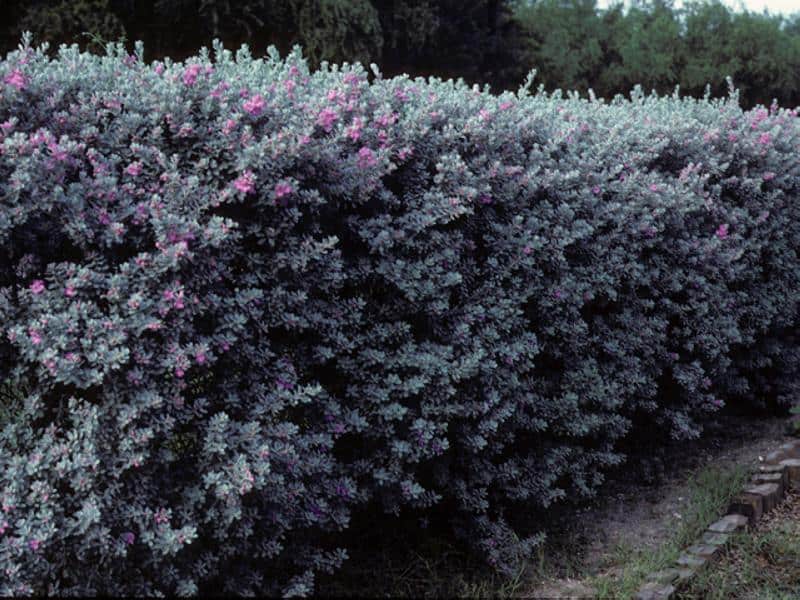The photograph depicts a well-trimmed, six-foot-tall hedge that extends out of frame, giving the impression of an endless green wall. The hedge features dark green leaves interspersed with sparse, dark purple flowers, resembling a lavender shrub. This dense foliage stands in front of taller green trees, which form a natural backdrop. The ground immediately in front of the hedge is lined with a small stone path, adding a neat border to the scene. The image appears aged, enhanced by a filter that imparts a dated, vintage look. Despite the presence of grass, the focus remains on the meticulously maintained hedge and its floral accents, with very little else visible in the close-up shot.